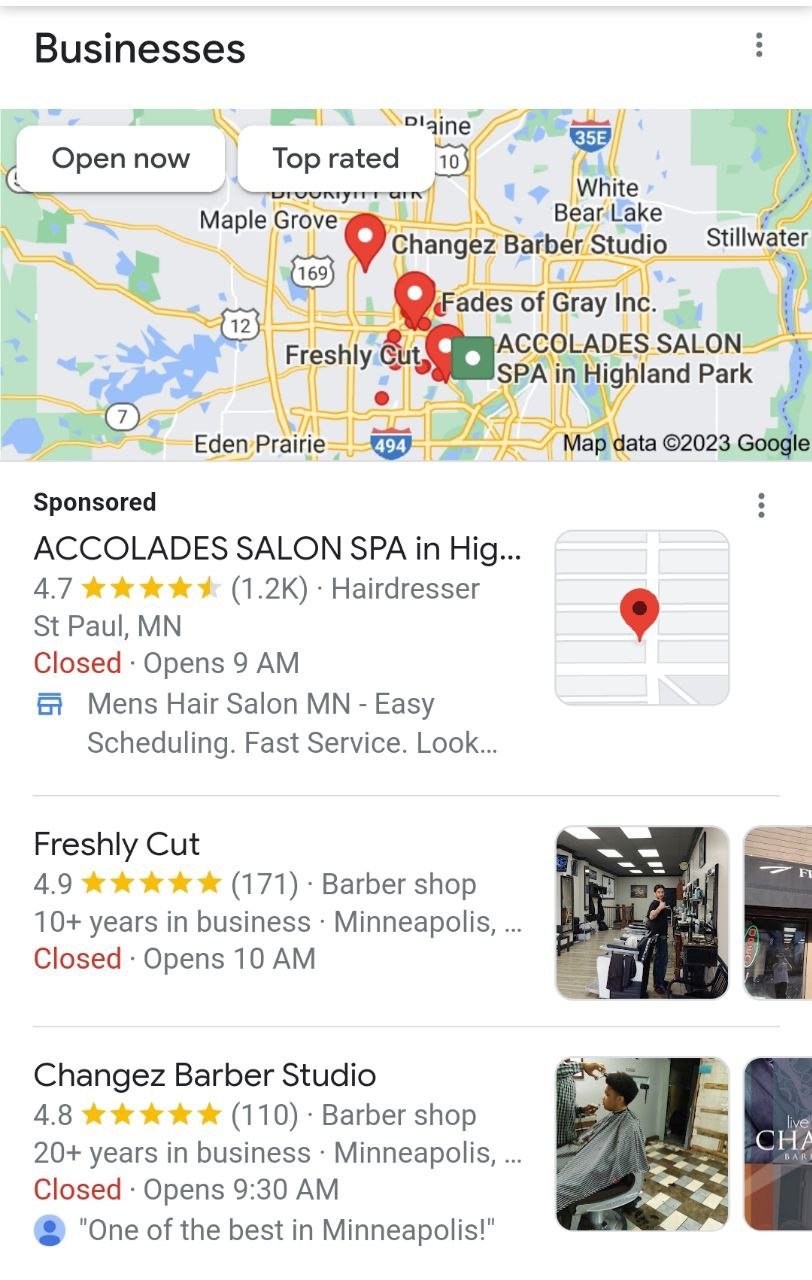This is a search result listing for spas and barbers in Highland Park, displayed in response to a search query. At the top of the listing, there's an interactive map allowing users to filter by "Open Now" and check the top-rated establishments. The listing highlights three businesses:

1. **Accolade Spa**: Rated at 4.5 stars, this establishment provides various spa services.
2. **Men's Hair Salon**: Known for its easy scheduling and fast service, this salon caters specifically to men.
3. **Freshly Cut**: This barbershop has earned a perfect 5-star rating, boasts 10 years of operation, and is located in Minneapolis.
4. **Train Jez Barber Studio**: Holding a stellar 5-star rating, this barbershop has over 20 years of experience and is also based in Minneapolis. Recognized as one of the best in the city.

Each entry offers detailed information, including ratings and years in business, helping users make informed choices.